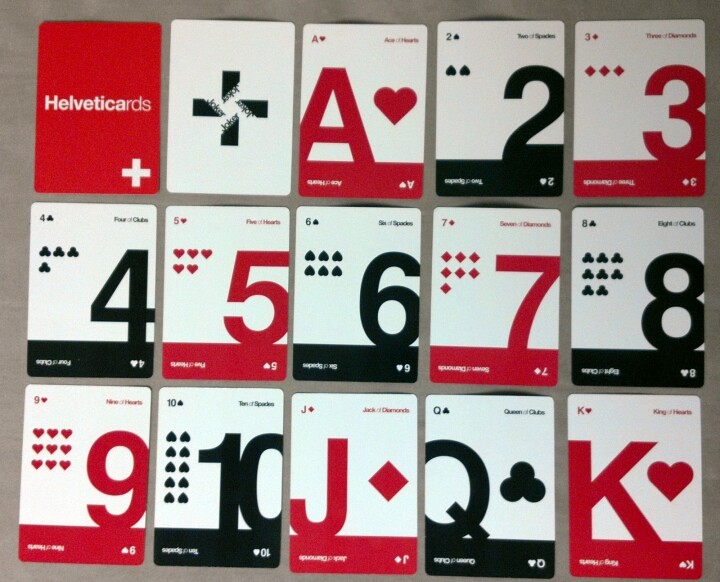In the image, there are three rows of five playing cards, totaling 15 cards, arranged in a front-facing perspective. Each row displays a variety of cards with distinct characteristics and designs. 

- **Top Row, from Left to Right:** 
  - The first card is a red card featuring the text "HELVETICARDS" with a white cross in the bottom right corner. 
  - The second card is white with a black cross. 
  - The third card is the Ace of Hearts, displaying a large "A" and a red heart beside it.
  - The fourth card is the Two of Spades, which has a black "2" and two black spades below it.
  - The fifth card is the Three of Diamonds, showing a large red "3" with three red diamonds and a red background.

- **Middle Row, from Left to Right:**
  - The first card is the Four of Clubs, featuring a black "4" on the right and four black clubs on the left.
  - The second card is the Five of Hearts, showing a large red "5" with five red hearts beside it.
  - The third card is the Six of Spades, displaying a large black "6" and six black spades to the left.
  - The fourth card is the Seven of Diamonds, displaying a red "7" with seven red diamonds.
  - The fifth card is the Eight of Clubs, featuring a large black "8" with eight black clubs.

- **Bottom Row, from Left to Right:**
  - The first card is the Nine of Hearts, showing a large red "9" and nine red hearts beside it.
  - The second card is the Ten of Spades, displaying a large black "10" with ten black spades.
  - The third card is the Jack of Diamonds, featuring a "J" and a red diamond.
  - The fourth card is the Queen of Clubs, showing a "Q" with black clubs.
  - The fifth card is the King of Hearts, displaying a "K" along with a red heart.

All cards share a consistent light gray background, which helps unify their presentation.